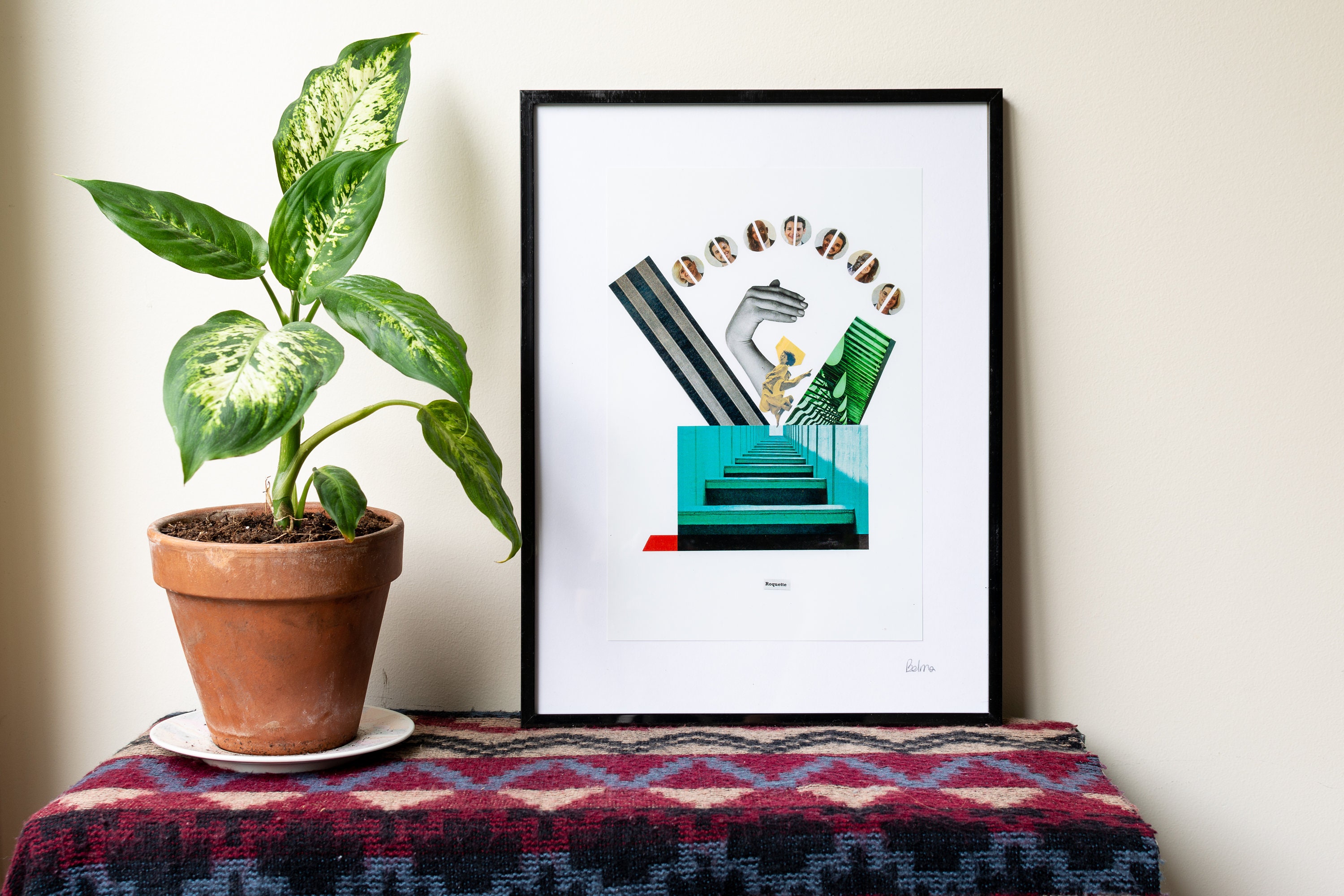This is a detailed product image of a framed poster displayed in a carefully curated setting. The poster, encased in a thin black frame, features an abstract collage on a white background. Prominently, it includes blue steps against a matching wall, a lady in yellow dancing, and several half-circles each showing split images of different people. The collage is complemented by black and white striped lines and additional abstract elements, including an image of a hand and parts of an arm. 

The framed poster is set against a cream-colored, off-white wall with subtle shadows, enhancing the artistic ambiance. It rests on a table draped with a Southwestern-style blanket adorned with blue, black, gray, maroon, and cream-colored stripes, adding a rustic flair. To the left of the poster, there is a large potted plant in a brown terracotta pot placed on a white dish. The plant features lush green leaves with white or cream-colored variegation, contributing to the overall aesthetic appeal of the image.